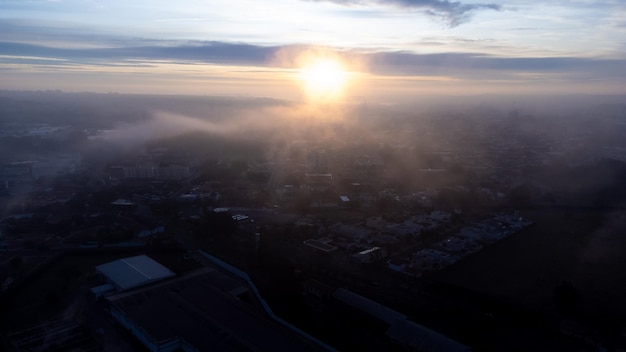In this photograph, captured in a landscape layout from an elevated vantage point, possibly from a window seat inside an airplane, we witness a mesmerizing scene of a sun either rising or setting. Dominating the top half of the image is a vibrant blue sky, subtly veiled by patches of gray, hazy clouds. At the center, slightly below the sky's zenith, sits a radiant white sun, its rays transitioning gracefully from bright white to hues of orange and pink. The light bathes the surrounding clouds and sky in an ethereal glow. Below this celestial display, the landscape becomes indistinct and dark, with faint, blurred outlines that suggest rooftops or a gated community, shrouded in a misty fog or smog. The fog, illuminated by the sun, appears to drift serenely from left to right, adding a mystical quality to the scene. The horizon delineates the boundary between the luminous sky and the shadowy earth, creating a captivating contrast that makes this sunrise or sunset a focal point of serene beauty.